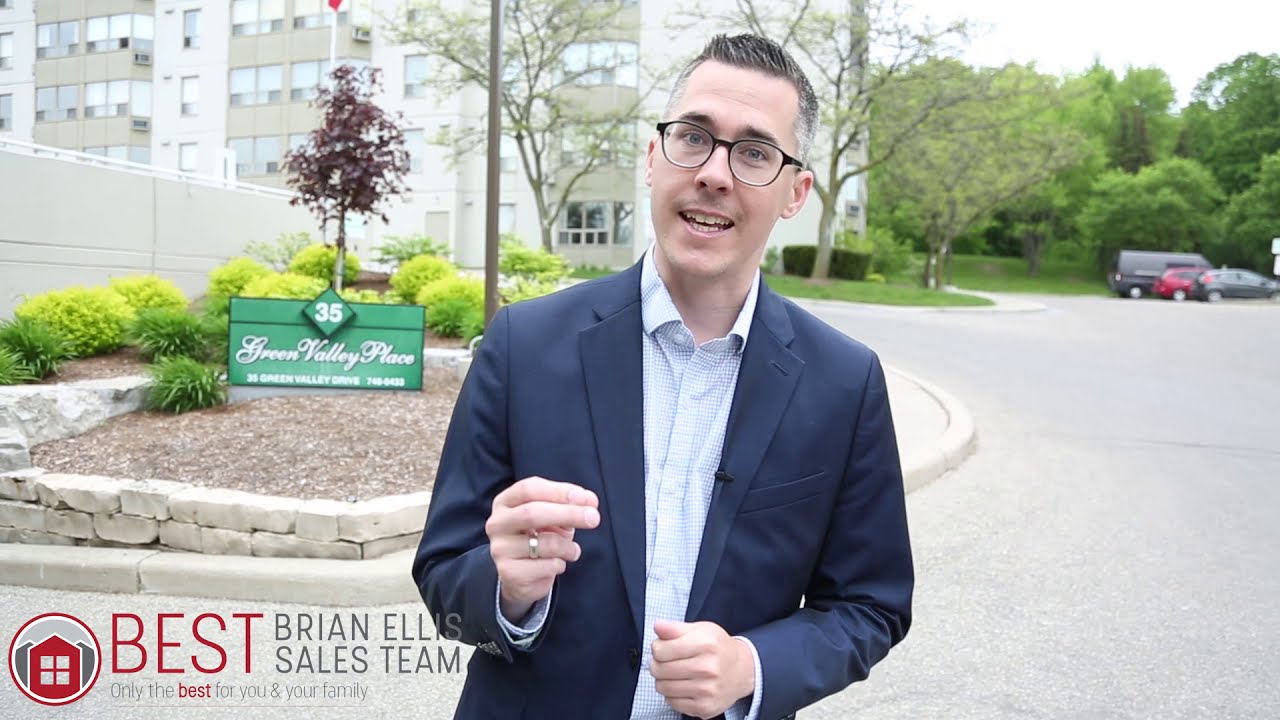In the image, a middle-aged, Caucasian man stands in the center, dressed in a blue sports coat and an unbuttoned light blue button-up shirt, collar slightly raised. He wears black-rimmed glasses and his head tilts slightly to the right. His right-hand is raised in a gesture, displaying a gold ring on his ring finger, while his left hand rests clenched near his stomach. Directly behind him, a green sign reads "35 Green Valley Place," with indistinct white lettering beneath it. 

To the left of the sign is a circular red logo featuring a red house and the words "Best Brian Ellis Sales Team, Only the best for you and your family" in gray letters, with "best" highlighted in red. The background showcases a multi-story building brimming with windows, flanked by trees and shrubs. One tree has purple leaves, while another is sprouting green leaves. A parking lot on the right contains three vehicles—a van and two sedans—and behind them, dense, dark green trees obscure the view. The scene, imbued with various shades of green, red, tan, white, maroon, and gray, captures an outdoor setting under a white sky, likely depicting a real estate advertisement mid-day.